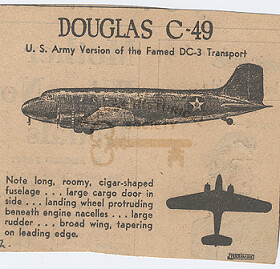The image is a digitized monochrome page, likely from a vintage newspaper or magazine, featuring detailed information about the Douglas C-49, the U.S. Army version of the famed DC-3 transport aircraft. At the top of the page, bold text reads, "Douglas C-49, U.S. Army version of the famed DC-3 transport." Beneath this heading, there is a black and white photograph of an old-fashioned propeller plane, showcasing its long, cigar-shaped fuselage, large cargo door on the side, landing wheels protruding beneath the engine nacelles, a sizeable rudder, and broad wings tapering on the leading edge. Below the photograph, there is a simple black outline of probably the same aircraft viewed from either the top or the bottom. Notably, the image also includes a watermark in the middle, featuring a faint, yellowish old-fashioned skeleton key. Additionally, on the side of the plane, there's an emblem of a star inside a circle. Lastly, a small, rectangular text section at the bottom provides further details about the plane’s design and functionality.